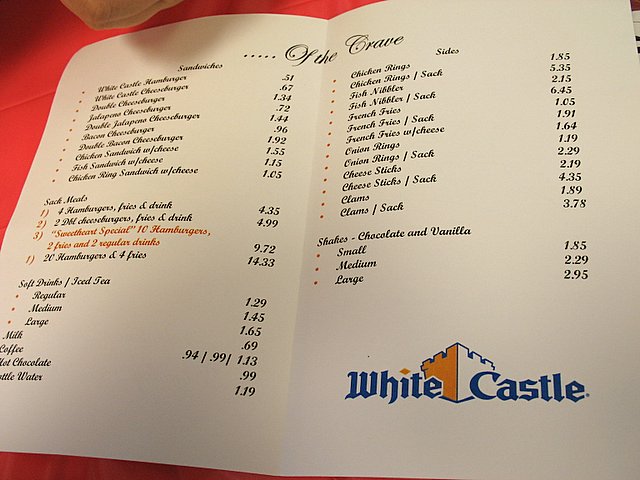This image captures an old paper menu from the restaurant White Castle, prominently placed on an orange table. The menu itself features a clean design with "White Castle" inscribed in blue on a white background, accompanied by an illustration of a castle, colorfully split with one half in yellow and the other half in white. Titled "Of the Crave" at the top, this nostalgic menu highlights a White Castle hamburger priced at just 51 cents, a clear indicator of its vintage origin. 

The menu lists various items, including a cheeseburger for 67 cents and a jalapeño cheeseburger for 72 cents. Combos such as four hamburgers, a fry, and a drink are priced at $4.35. Soft drink options range from $1.25 to $1.65, scaling up from regular to large sizes. Milkshakes in both chocolate and vanilla flavors are available, with prices ranging from $1.85 for a small to $2.95 for a large. Additionally, the menu offers side orders like chicken rings, onion rings, and cheese rings, each detailed with its respective price, reflecting a simpler pricing era. This menu serves as a charming relic from a bygone time, evoking memories of past dining experiences at White Castle.